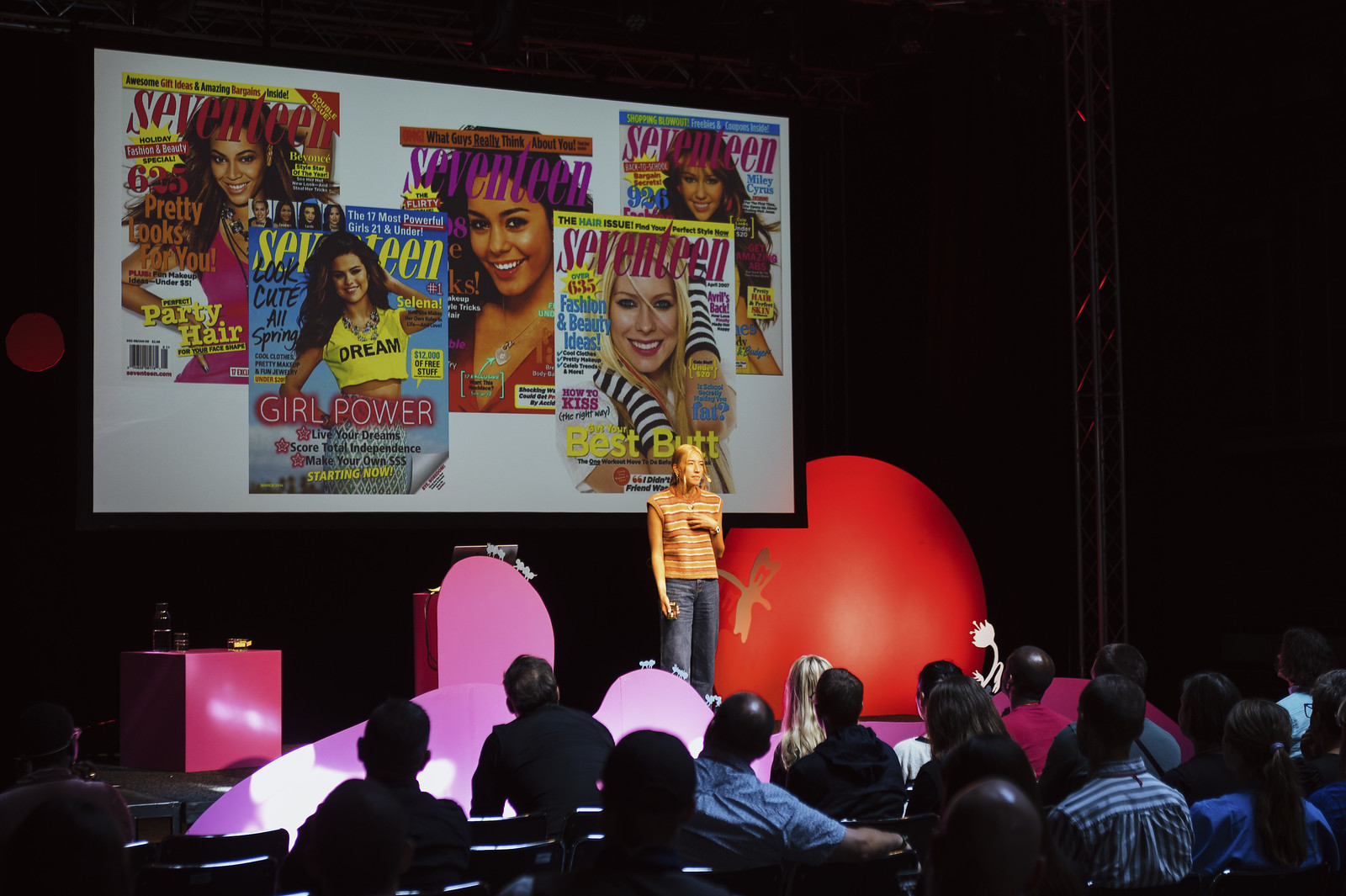In this indoor conference setting, a woman takes the stage, addressing an attentive audience seated before her. She wears blue jeans and a short-sleeved, orange-brown blouse, and has blonde or perhaps blondish-reddish hair. The stage around her is decorated with various geometric shapes: a large pink cube to the far left, a pink oval directly behind her, and a substantial red circular shape to her right. Above her, a screen prominently displays five covers of Seventeen magazine, each one featuring a young woman and adorned with colorful, bright lettering. The magazines are arranged in a staggered fashion, with three in the background and two in the foreground, suggesting the woman's association with or representation of the magazine.